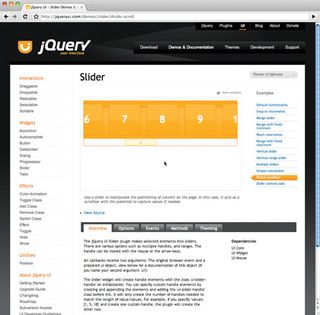The image is a detailed screenshot of the JQRY website, spelled J-Q-U-E-R-Y, prominently displayed in the top left-hand corner. The screenshot reveals that the site is being accessed on an Apple computer, as evident by the red, yellow, and green circles in the top left-hand corner of the browser window. This browser only has one active tab, highlighting the JQRY website.

Centrally featured at the top of the webpage is an orange slider, resembling a belt, displaying a range of white numbers from 6 to 10. Below this slider, the site offers various descriptions and information. On the left side, there is a navigational menu listing clickable items, while on the right side, there are links in blue text providing additional resources.

The top section of the website is black and contains several important navigation links, including "Download" and "Preview." The overall layout suggests a well-organized interface designed for efficient navigation and access to information.